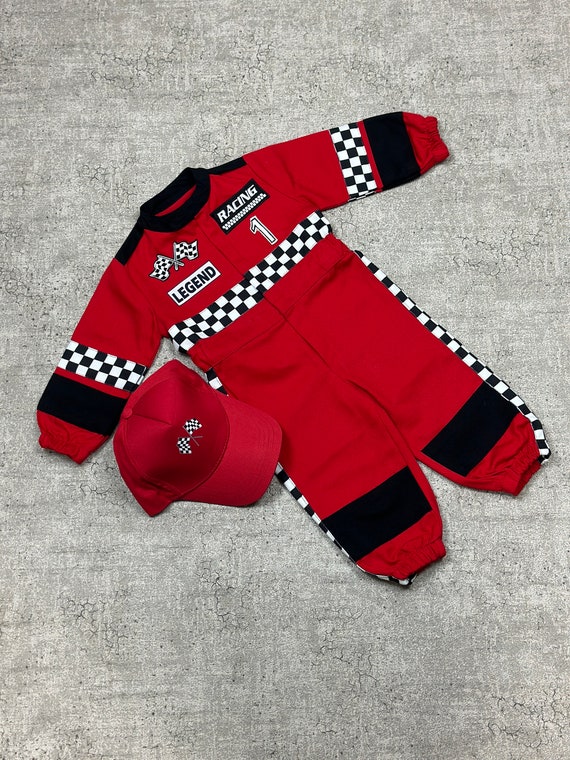The image displays a small child's red racing-themed onesie laid out on a cracked, gray concrete surface. The onesie, designed to resemble a racing jumpsuit, features black and white checkered print across the chest, down the sides of the legs, and along the arms. There are additional black stripes at the collar, wrists, and ankles. The uniform is adorned with several patches, including one that reads "Racing," another that says "Legend," and a prominent "Number One" alongside two crossed checkered flags on the right lapel. Accompanying the onesie is a matching red baseball cap, also featuring two crossed checkered flags on the front. Notably, the cap appears significantly larger, possibly sized for an adult rather than the child who would wear the onesie.